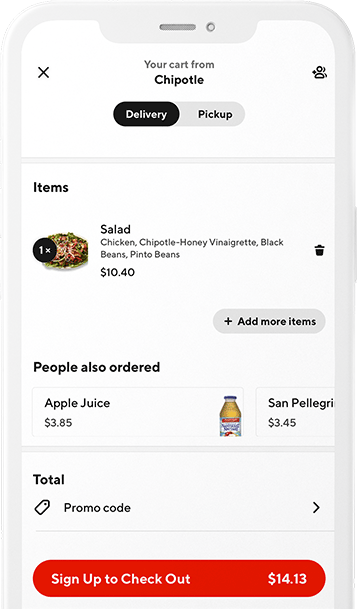**Caption:**

A detailed image of a mobile phone screen displays a Chipotle online order under the category of websites. At the top, the screen shows the title "Your Cart" from Chipotle, and beside it is a small figure icon and an 'X' button for closing. The delivery option is selected above a list of items. The cart contains one item: a salad with chicken, Chipotle Honey Vinaigrette, black beans, and pinto beans priced at $10.40. A trash can icon next to the item allows for deletion.

An option to add more items is provided below the listed order. Additionally, there's a suggestion section with images, where "People also ordered" apple juice for $3.85 and San Pellegrino for $3.45 are highlighted. The total cost is indicated at the bottom, accompanied by a space for entering a promo code. Beneath this, a red bar with white text prompts users to "Sign up to checkout." The final total is $14.13. Though small, the images of the items in the order, including the salad and apple juice in a glass bottle with a blue lid, are shown.